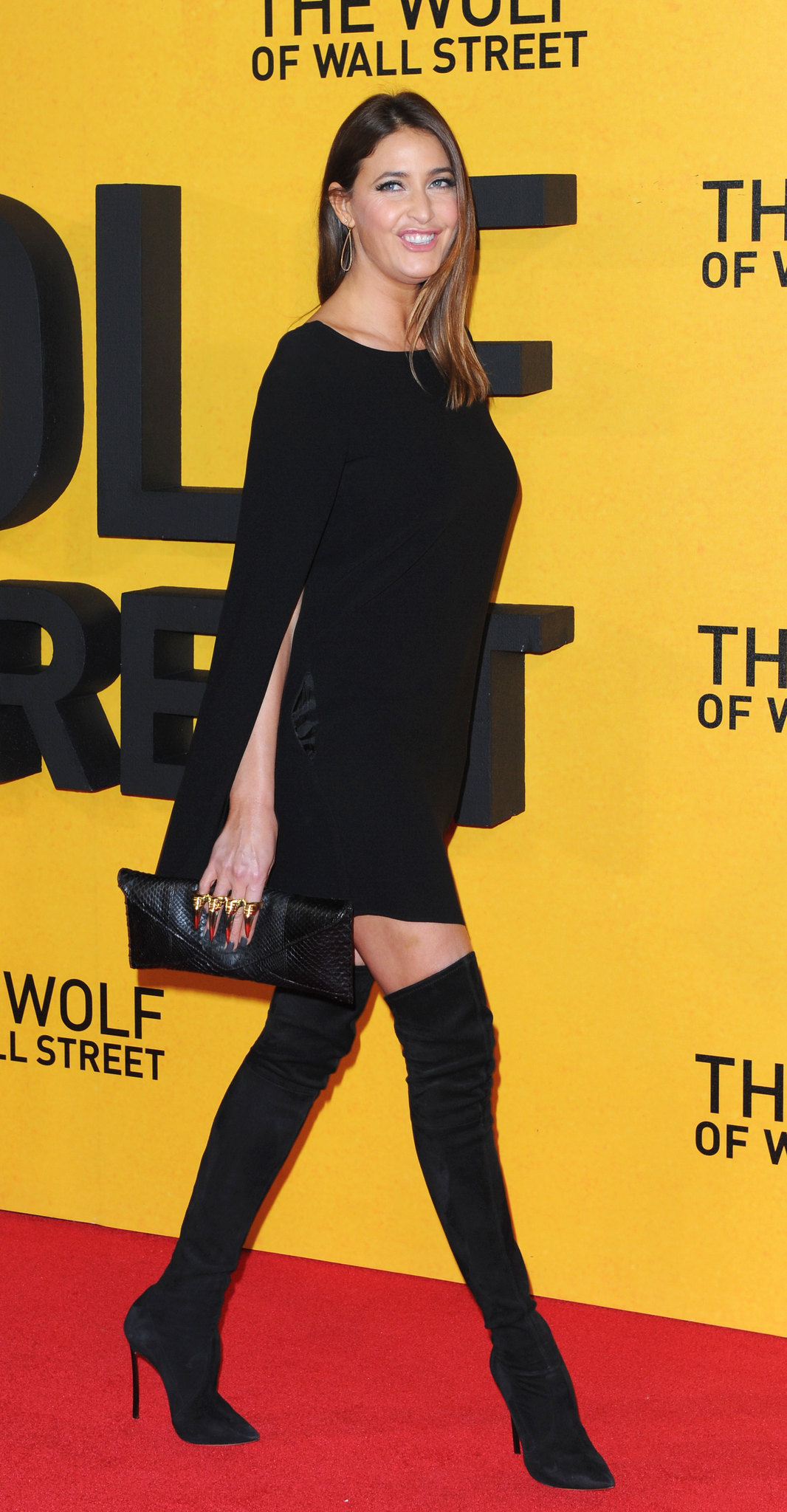The photograph captures a woman, possibly in her 30s or 40s, who has light to medium brown, shoulder-length hair, standing and smiling on a red carpet event, likely for a movie premiere. She is wearing a stylish, long-sleeved black dress that ends mid-thigh, paired with thigh-high black boots. In one hand, she holds a black clutch bag, and she accessorizes with several golden rings. The backdrop is a distinctive yellow wall adorned with black text repeatedly stating "The Wolf of Wall Street," indicating the likely occasion for the photograph. The woman exudes confidence and elegance as she showcases her ensemble.